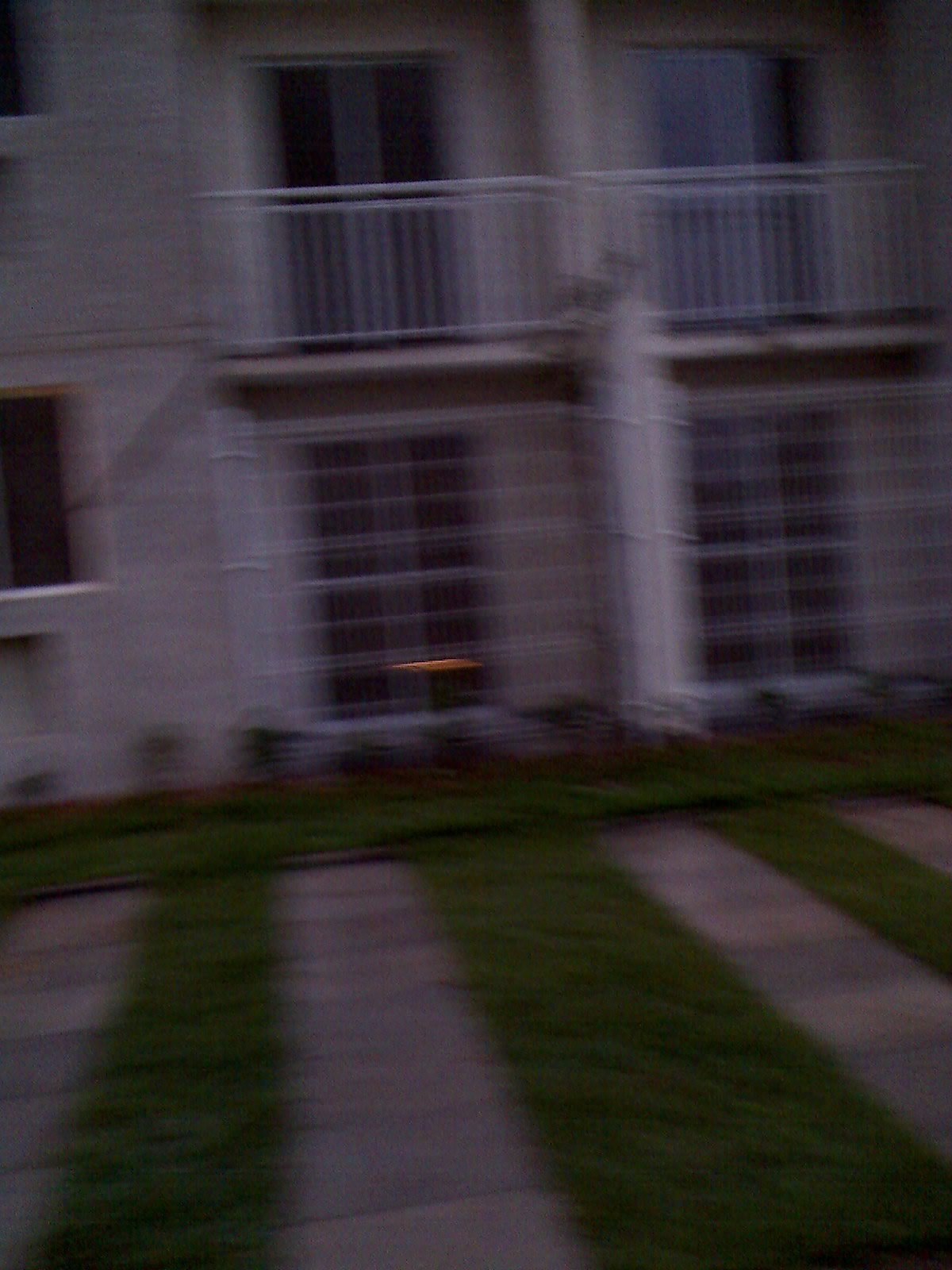The image depicts a slightly blurry view of a two-story apartment complex. The lower level features several windows and a small porch area bordered by a low wall and flanked by bushes. Directly above, on the second floor, there are sliding glass doors with white railings that lead to diminutive porches, each separated by a wall. To the left of the structure, white blocks or bricks are visible. In the foreground, alternating stripes of grass and concrete blocks extend towards the viewer, suggesting this could be a parking area, although currently, it is devoid of any parked vehicles.